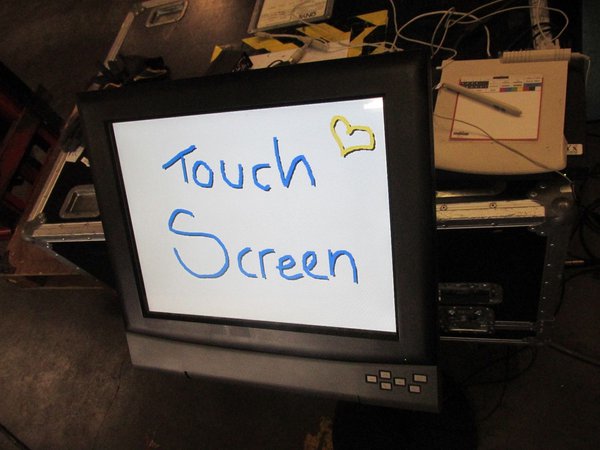The photo depicts an electronic setup centered around a touchscreen monitor device. The monitor, encased in black, displays a white background with the word "touchscreen" handwritten in blue digital ink. The word "touch" is positioned at the top and "screen" at the bottom. A yellow outline of a heart is visible in the upper right corner of the screen. This setup is situated on a sturdy industrial-type black and silver metal box, likely used for carrying electronic equipment. Resting on top of this box is a white electronic signing pad, equipped with a corded digital pen. In the background, various other electronic components and wires are scattered, adding to the complex array of devices in the scene. The overall environment suggests a workspace filled with interconnected electronic tools and instruments.